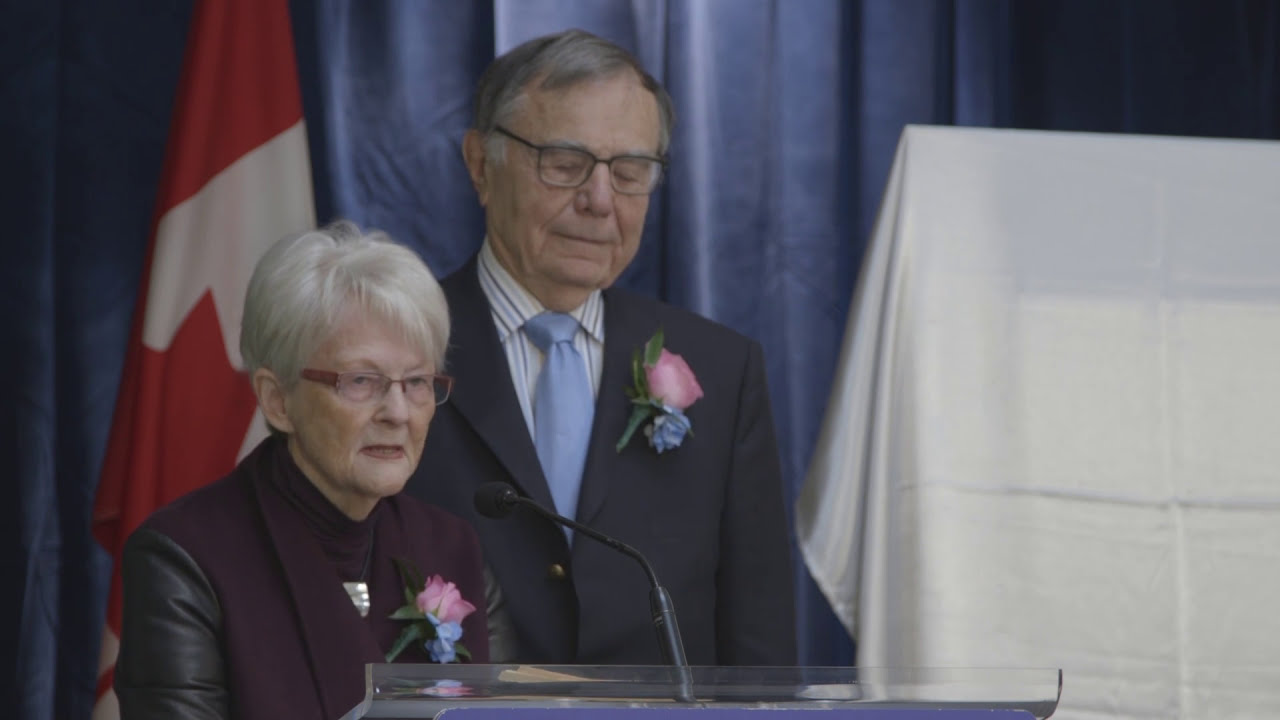In this image, an older man and woman are standing on a stage adorned with a long blue curtain and a red and white flag, possibly Canadian, though it is partially obscured by the way it hangs on a pole. The woman, dressed in a black suit with pink glasses and white hair, stands at a podium with a microphone close to her mouth. She wears a pink and blue floral boutonniere. The man, positioned just behind her left shoulder, sports a blue suit, a light blue tie, and a white and blue striped shirt; he also wears the same pink and blue boutonniere. Off to the right side of the stage, a white sheet covers a square-shaped object, adding to the dignified yet mysterious ambiance of what appears to be a formal or memorial service.